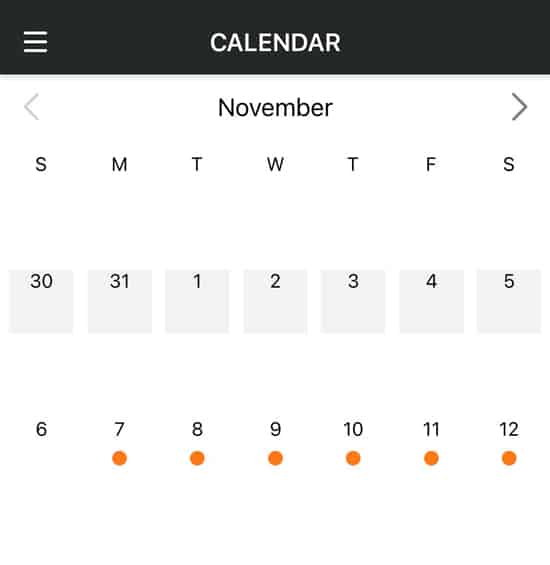The image is a screenshot of a digital calendar displayed within a mobile app interface. At the top, a black bar featuring white text includes a menu button, represented by three horizontal lines, and the title "CALENDAR" in all capital letters. Below this header, the main calendar interface spans the majority of the screen with a clean, white background and black text. The visible month is November, beginning on a Tuesday, with the last two days of October, the 30th and 31st, appearing in the initial rows.

The calendar is organized in a standard format with weeks beginning on Sunday and ending on Saturday, each day occupying its column. Notably, no events are marked until the week of November 7th through November 12th, where individual activities are indicated by small orange dots. These dots suggest multiple separate events rather than continuous occurrences, as the calendar lacks a connecting bar that would typically indicate a multi-day event. This straightforward calendar setup exemplifies a basic scheduling layout likely common to tablet or smartphone applications.